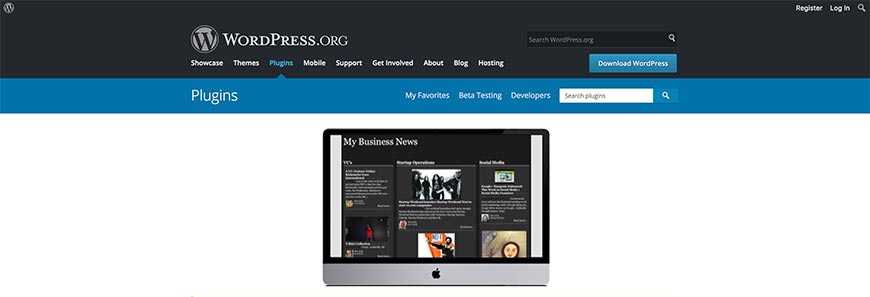The image showcases a WordPress.org webpage. In the top left corner, there is a small WordPress logo, featuring a 'W' within a gray circle, encircled by a black ring and another gray ring. This logo appears multiple times across the page. Adjacent to the logo, to the right, the text "WordPress.org" is prominently displayed in white, with 'WordPress' in capital 'W' and 'P', and 'ORG' in all caps, set against a black background. Nearby, there is a search bar labeled "Search WordPress.org" with a white magnifying glass icon.

A blue "Download WordPress" button with white text is also visible. In the top right-hand corner, there are links for "Register" and "Login", as well as another magnifying glass icon for the search functionality.

The main navigation menu, set just below the top section, includes links labeled "Showcase," "Themes," "Plugins," "Mobile," "Support," "Get Involved," "About," "Blog," and "Hosting." This illustration focuses on the "Plugins" section, as indicated by a blue triangle pointing upwards towards the "Plugins" menu item. Beneath this, the word "Plugins" appears again in white text inside a blue rectangle.

Another navigation bar includes links labeled "My Favorites," "Beta Testing," and "Developers," along with a white search bar that reads "Search Plugins" and contains a blue magnifying glass icon.

The page content reveals that the "Plugins" page is active. Below this, the image features a picture of an Apple computer screen displaying a section titled "My Business News," which includes six tiles, each featuring different headlines.